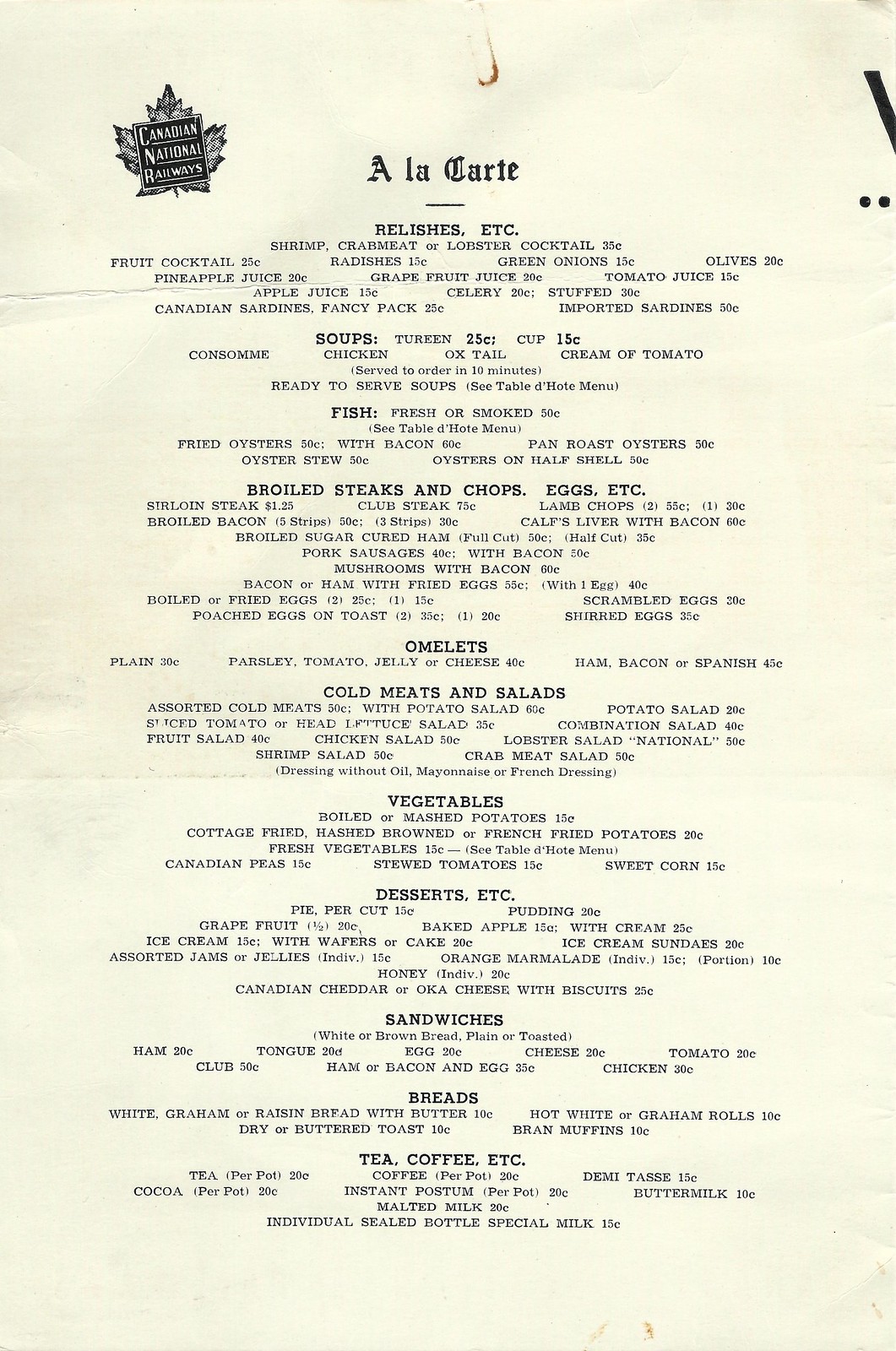This image displays an extensive à la carte menu. At the top, it prominently features the title "À la Carte." The menu is divided into various sections, each offering a range of culinary delights. Under "Ready Relish, etc.," options include shrimp, crab meat, or lobster cocktail, fruit cocktail, radishes, green onions, olives, pineapple juice, grapefruit juice, and tomato juice. There are also options for Canadian sardines and fancy pack imported sardines.

The next section, "Soup," lists several varieties such as terrine, cup, consomme, chicken, oxtail, and cream of tomato, with a designation for ready-to-serve soup. The "Fish" section offers choices of fresh or smoked fish, fried oysters with bacon, and pan-roast oysters.

Moving on to "Steaks and Chops", options include boiled, sirloin steaks, cups, and lamb chops. The menu also features "Eggs, Etc." and an assortment of cold meats accompanied by potato salad. Simple offerings like potato salad and sliced tomatoes are also included.

Finally, the menu transitions into sections for "Vegetables," "Desserts," and "Sandwiches," hinting at a broad array of items available. Overall, this menu features a diverse selection of dishes catering to a variety of tastes and preferences.